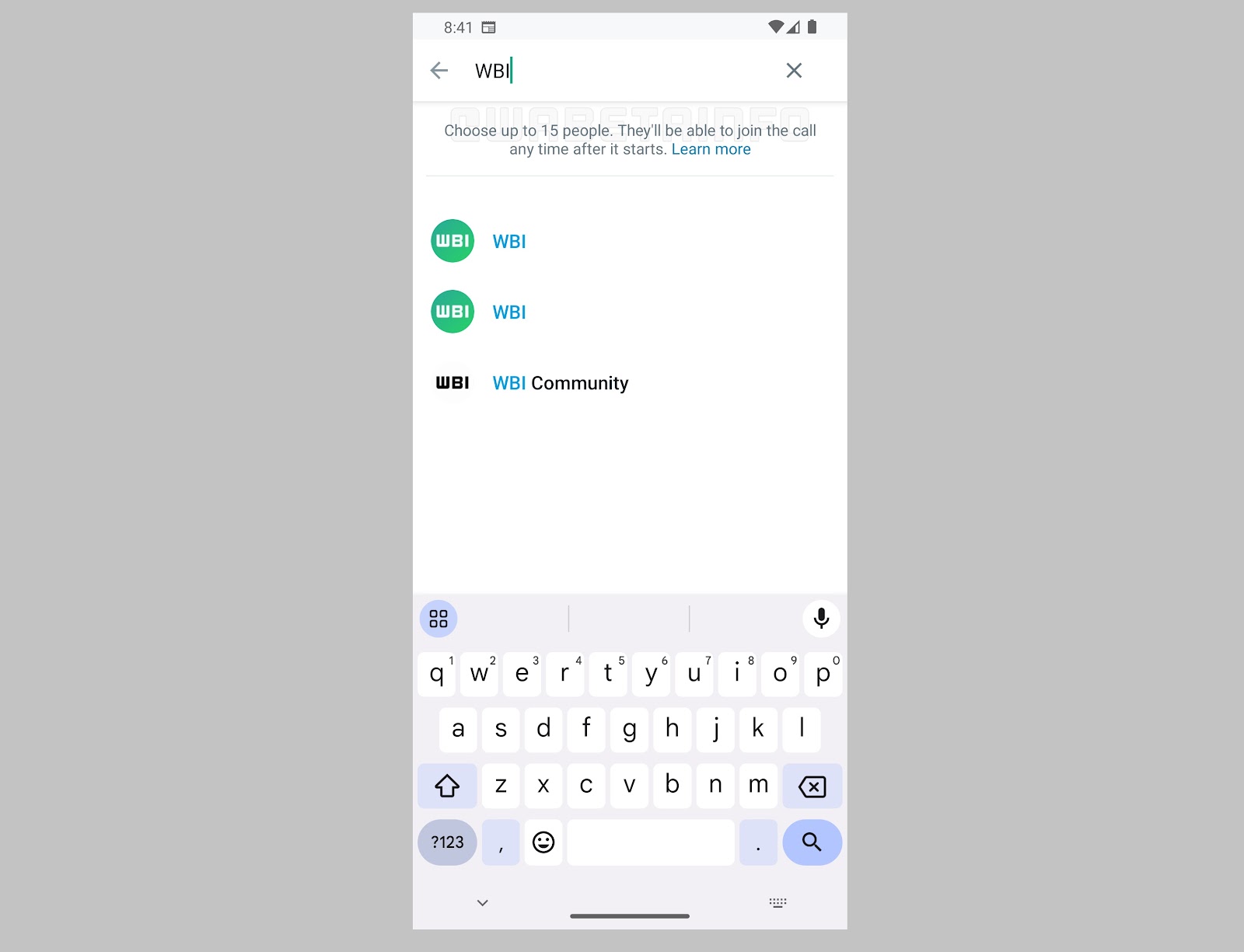**Detailed Caption:**

The image showcases a complex interface against a solid gray background. 

- **Top Section:** It begins with a light white rectangular section that contains a set of indicators and icons. At the top left, "8:41" is displayed alongside a calendar icon. Adjacent to these elements is an image icon. Towards the far right of this section, battery status shows full charge and the Wi-Fi signal indicates full connectivity.

- **Middle Section:** Below the top indicators, a navigation bar features a left arrow, the acronym "WBI" marked in green, a spacer line, and a close 'X' button on the right. The next line down presents an instruction in light black font: "Choose up to 15 people that will be able to join the call." Beneath in a greenish font is a hyperlink text: "Learn more."

  A gray divider line follows, separating the instruction from the subsequent navigation options. On the left, "WBI" appears in a green circle, succeeded by "WBI" in blue text. This pattern repeats: "WBI" in a green circle, "WBI" in blue, then "WBI" in black, followed by "WBI" in blue again, and finally, the word "Community" in black.

- **Bottom Section:** This section transitions back to a gray background. On the left, there’s a light blue tile with four smaller squares inside it. To the right sits a black microphone icon. Nearby, a virtual keypad with white keys and light black numbers includes: 1, 2, 3, 4, 5, 6, 7, 8, 9, and 0. 

  Additional navigational elements include arrows. A black outlined arrow points up on the left, and another arrow points left towards an 'X'. There’s also a numeric and punctuation pad below, featuring keys like "123" and a question mark, highlighted in light blue against a white background with black outlines. Symbols like a comma and a happy face are also present.

  To the right, there’s a magnifying glass icon enclosed in a blue circle, next to a search input box in black font. Finally, at the bottom, a separation is marked by a black horizontal line with a keyboard icon on the right and a down arrow on the left, indicating additional functions or a menu expansion.